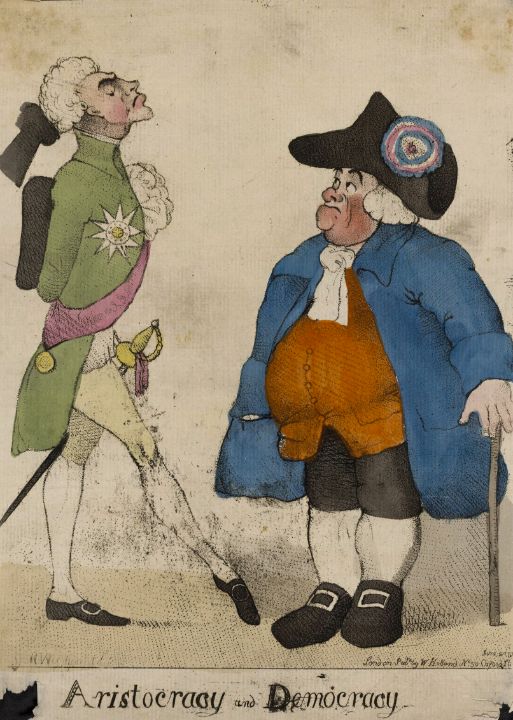The image is a detailed, old cartoon, likely from the late 1800s or earlier, depicting two men representing contrasting societal roles of the time, labeled "aristocracy and democracy" in black letters at the bottom. The paper looks aged with some torn parts at the bottom edge.

On the right side stands a shorter man reminiscent of Napoleon or Benjamin Franklin. He is quite portly, dressed in black shorts with white tights, and black shoes with silver buckles. He wears a large navy blue jacket over a mustard-colored shirt, complemented by a white scarf tied around his neck. His attire includes a powdered wig and a black hat adorned with a large blue and pink flower. The man holds a gray walking stick in his right hand.

The left side features a much taller and thinner man with a noble appearance. He dons a green military-style coat, decorated with a purple sash and a silver star. His right foot is poised daintily forward. He also wears white tights, black shoes with silver buckles, and carries a sword with a gold handle on his left side. His white powdered wig is tied with a black bowtie, and his hat sits slightly tilted as his chin is turned upward in a regal manner. 

An indistinct signature of the artist can be seen in the lower right-hand corner of the image.